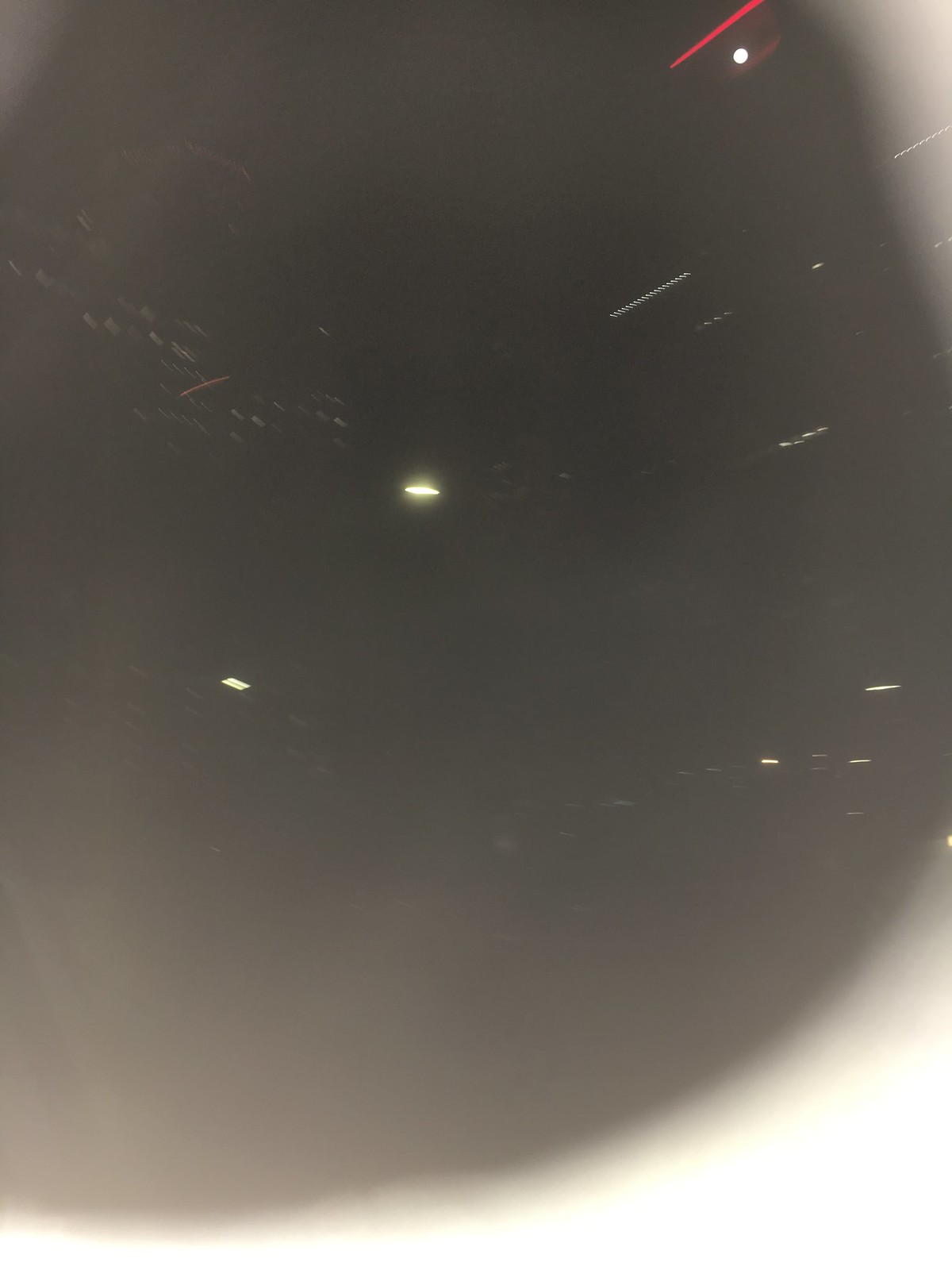This intriguing image appears to be captured in motion, resulting in a blurred and somewhat chaotic composition. Dominating the frame is a large, black circular blotch, which gradually fades into gray and white hues toward the edges of the picture. This central feature vaguely resembles a planet seen through a telescope, accentuated by a ring-like structure around it that is predominantly white.

Scattered throughout the image are white and red lines that streak across the scene, adding a dynamic, almost ethereal quality to the photograph. On the left side, faint, light gray or white text emerges against the dark background, contributing an obscure, mysterious element to the overall composition.

Despite its apparent flaws as a photograph, the image holds a certain allure, perhaps inviting viewers to ponder its subject and the circumstances of its capture. The central planet-like object, coupled with the surrounding elements, hints at an astronomical observation, further emphasizing its unique and significant nature.